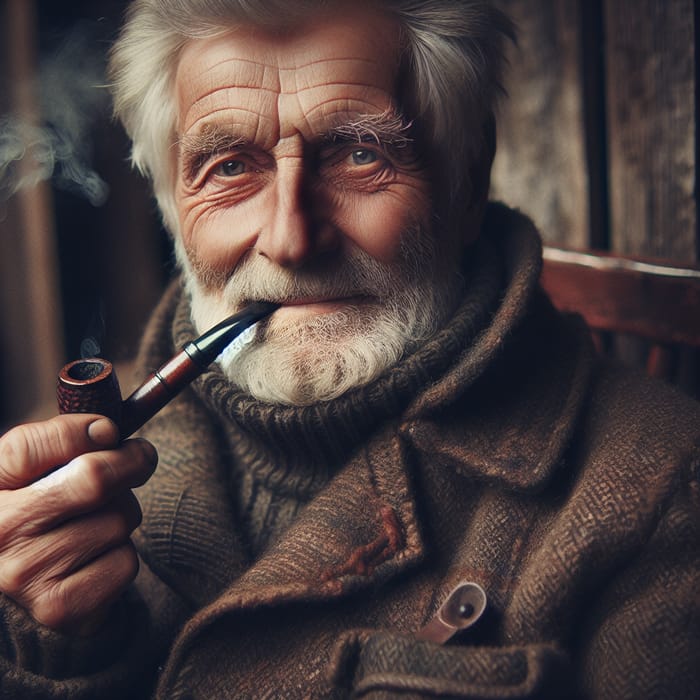In the image, an older gentleman with a full, pure white beard and mustache, as well as white hair, gazes directly at the viewer. He is seated in a wooden chair in front of a backdrop of darkened wooden planks, slightly out of focus but offering a rustic ambiance. His face is lined with wrinkles, and he has bushy gray eyebrows and striking green eyes that exude warmth and wisdom. Dressed for the cold, he wears a thick, cozy brown turtleneck sweater and a heavy, dark brown woolen coat. The man holds an old-fashioned wooden pipe in his hand, with disjointed smoke rising from it, hinting at the image's AI-generated nature due to its high resolution and certain unnatural details in the smoke. The overall impression is that of a debonair, seasoned gentleman, possibly in his late 50s, whose expressive eyes and gentle smile hint at a lifetime of stories and experiences.